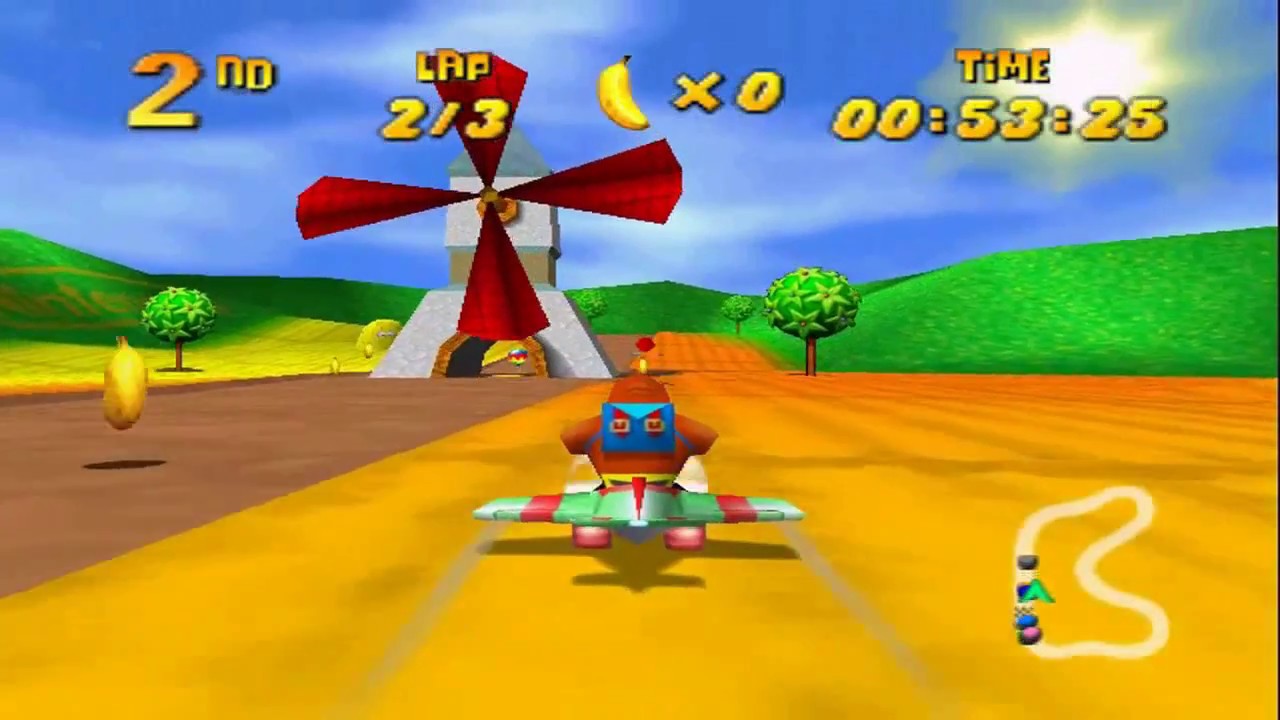The screenshot showcases a vibrant scene from a Nintendo 64 racing game, likely featuring the character Banjo from Banjo-Kazooie. Banjo is riding a small airplane on a dirt track surrounded by lush green fields, rolling hills, and a bright blue sky with scattered clouds and a prominent yellow sun. In the background, there's a windmill with red propellers, trees with star-shaped leaves, and a clear view of the racetrack. The top of the screen displays race details: the player is in second place, currently on lap 2 out of 3, with zero bananas collected. The race time is shown as 53.25 seconds. On the bottom right corner, a map illustrates the route with icons for different racers, showing Banjo and others progressing around the circuit, marked by colors like pink, light blue, dark blue, and grey.